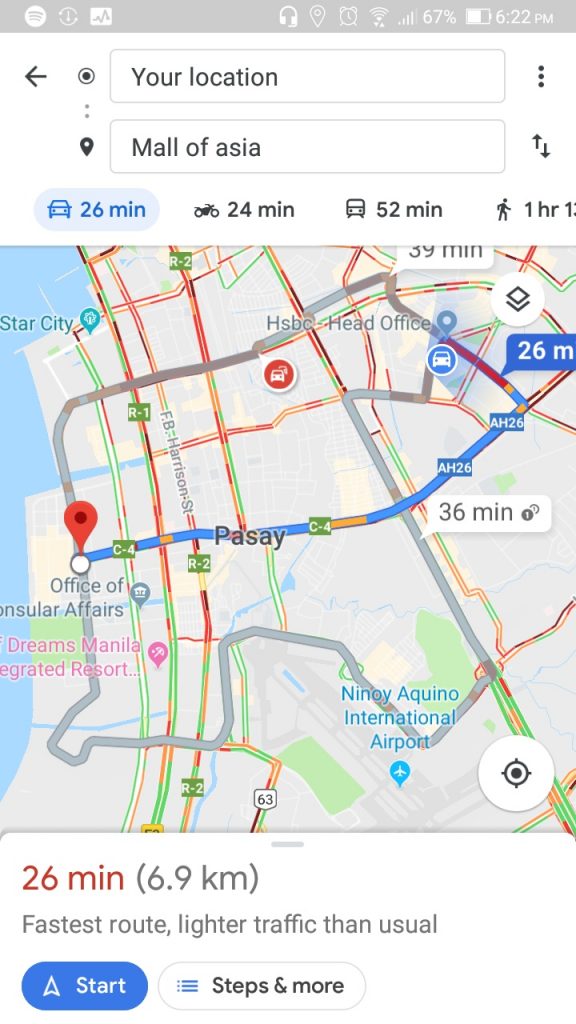**Detailed Caption:**

The screenshot appears to be from a mobile or tablet device, showcasing a navigation screen from Google Maps with detailed route information to the Mall of Asia. 

**Device Status Bar:**  
- At the top, there is a gray status bar presenting several icons from left to right: 
  - A potential Spotify icon.
  - Wi-Fi signal bars.
  - An information icon.
  - A bar graph. 
  - A pair of headphones.
  - A location tab.
  - An alarm clock. 
- The connectivity indicators show a full Wi-Fi signal and 4 out of 5 cellular network bars.
- The battery level is at 67%.
- The current time displayed is 6:22 PM.

**Google Maps Navigation Details:**
- There's an arrow pointing left adjacent to a black circle stating "Your location."
- To the right, three vertically aligned dots indicate further options.
- A location pin specifies "Mall of Asia" as the destination.
- Interactive arrows allow for switching route preferences.

**Route Information:**
- **By Car:** 26 minutes (highlighted in red), distance 6.9 kilometers, with a note indicating "fastest route, lighter traffic than usual."
- **By Motorcycle:** 24 minutes.
- **By Bus:** 52 minutes.
- **Walking:** Approximately 1 hour and 13 minutes.

**Navigation Interface:**
- A blue triangle button with white text labeled "Start" for initiating the route.
- An icon resembling a list with black text "Steps" and more options for route details.

The screenshot suggests someone is planning a journey from their current location to the Mall of Asia, with the car route selected as the fastest option.